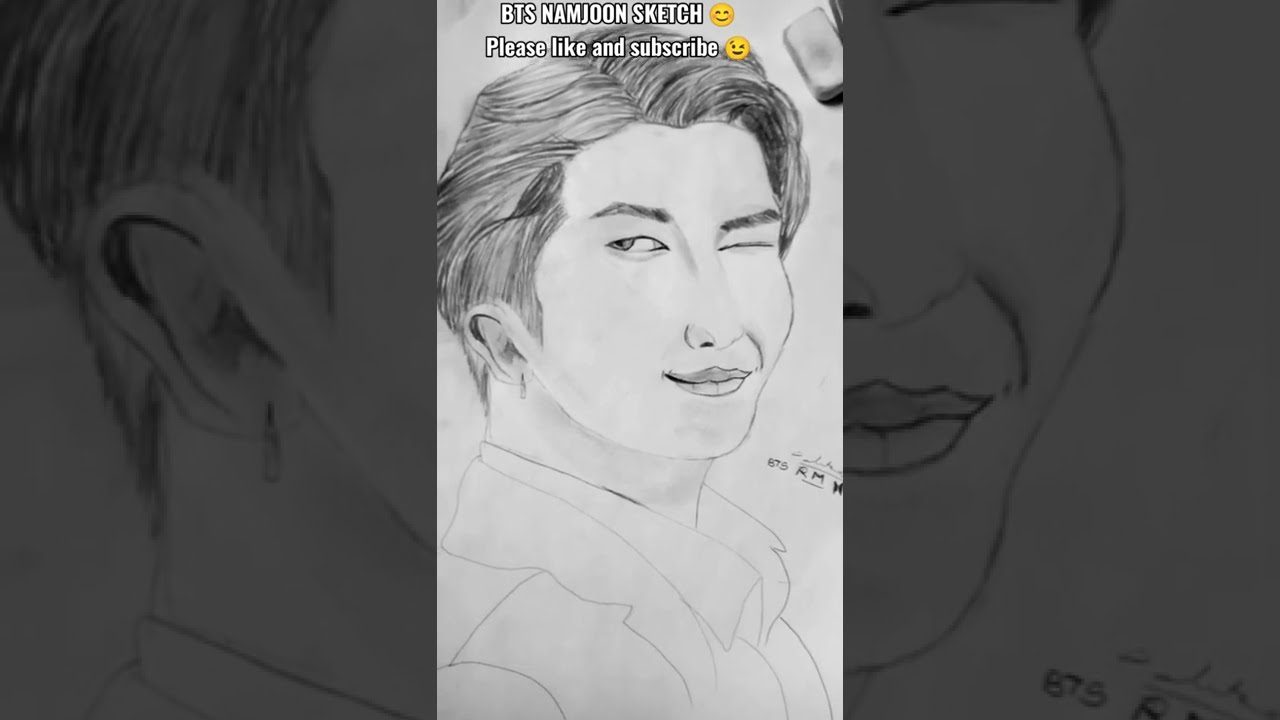The image showcases a pencil drawing of an Asian man, identified as BTS's Namjoon, prominently displayed in the center. The background features a darker, zoomed-in version of the same sketch, adding a shadowy border effect. At the top of the sketch, in white letters, it reads "BTS Namjoon Sketch" accompanied by a smiling emoji. Below this, the text "please like and subscribe" is followed by a winking emoji. Namjoon is depicted with parted, full hair that flops over to the right, suggesting a well-groomed look, possibly with gel. His facial expression is a wink, with his right eye closed and left eye open, paired with a slight smile that reveals a cheek dimple. He wears a white collared shirt, though minimal details of the shirt are sketched. The drawing is rendered in grayscale pencil, capturing the essence of the artist's hand-drawn style.